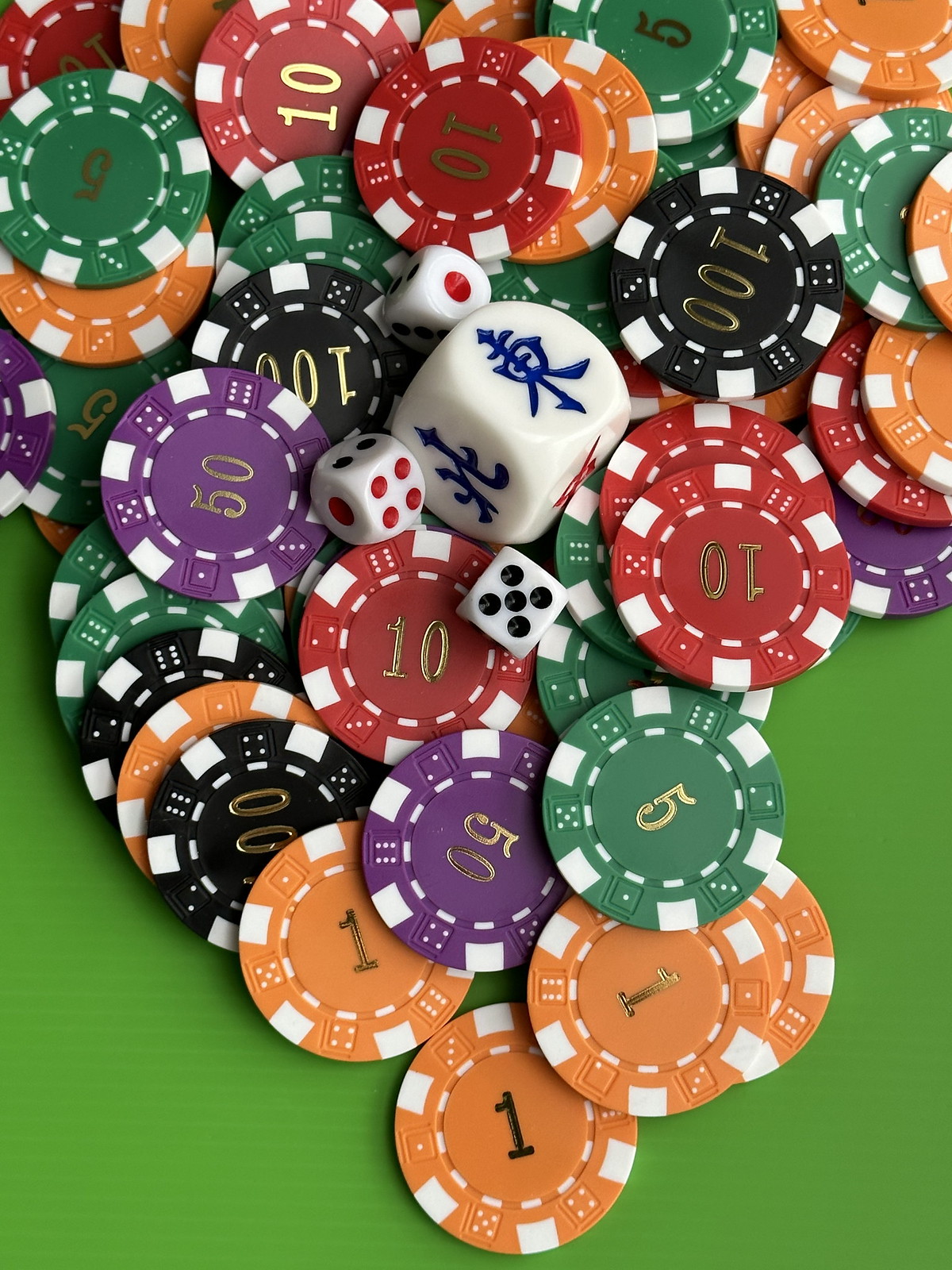The image showcases an array of colorful poker chips scattered haphazardly across a vibrant, pea green background, reminiscent of a casino setting. Dominating the scene at the center is a large, white die adorned with intricate Asian characters and navy blue designs, while one of its sides is distinctly marked with red printing. Surrounding the central die are three smaller, more conventional dice featuring red pips for the number one, navy pips for the number two, four, and five, with the number five prominently featuring black pips.

The poker chips themselves are a dazzling collection of orange, black, purple, and red, some glittering with golden accents as they catch the light. Each chip is clearly marked with its denomination: the black chips signify 100, the red chips denote 10, the green chips are worth 5, and the orange chips represent 1. This vivid ensemble of gaming paraphernalia fills the frame, creating a visually striking tableau.